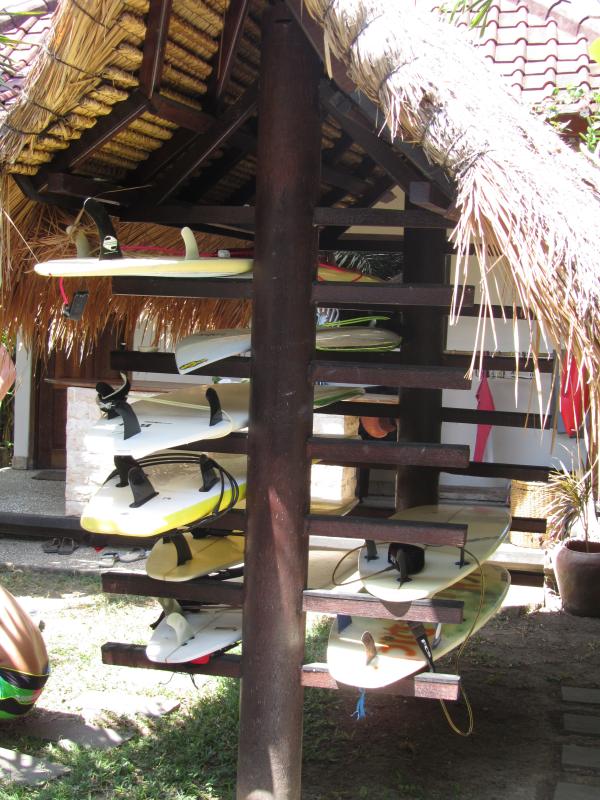This is an outdoor photograph of a surf shop or surfboard storage shack set in a well-lit tropical location, possibly illuminated by sunlight. The central structure features an A-frame roof made of bundled straw, designed to shield the area from sunlight. The shack includes a wooden rack with poles on either side and horizontal shelves extending upwards. 

On the left side of the rack, several surfboards are stored, wedged between the shelves, featuring various colors like white, yellow, and red, with some exhibiting painted graffiti. Each surfboard is secured with small locks. 

A total of 8 surfboards are visible, some positioned to show their fins. In the background, a boy sits on the grass, his back and part of his rump facing the camera. Another structure with an indistinct roof is partially visible further back in the scene, suggesting a beachside setting. The ground around the shack is covered in grass, further emphasizing the outdoor environment.